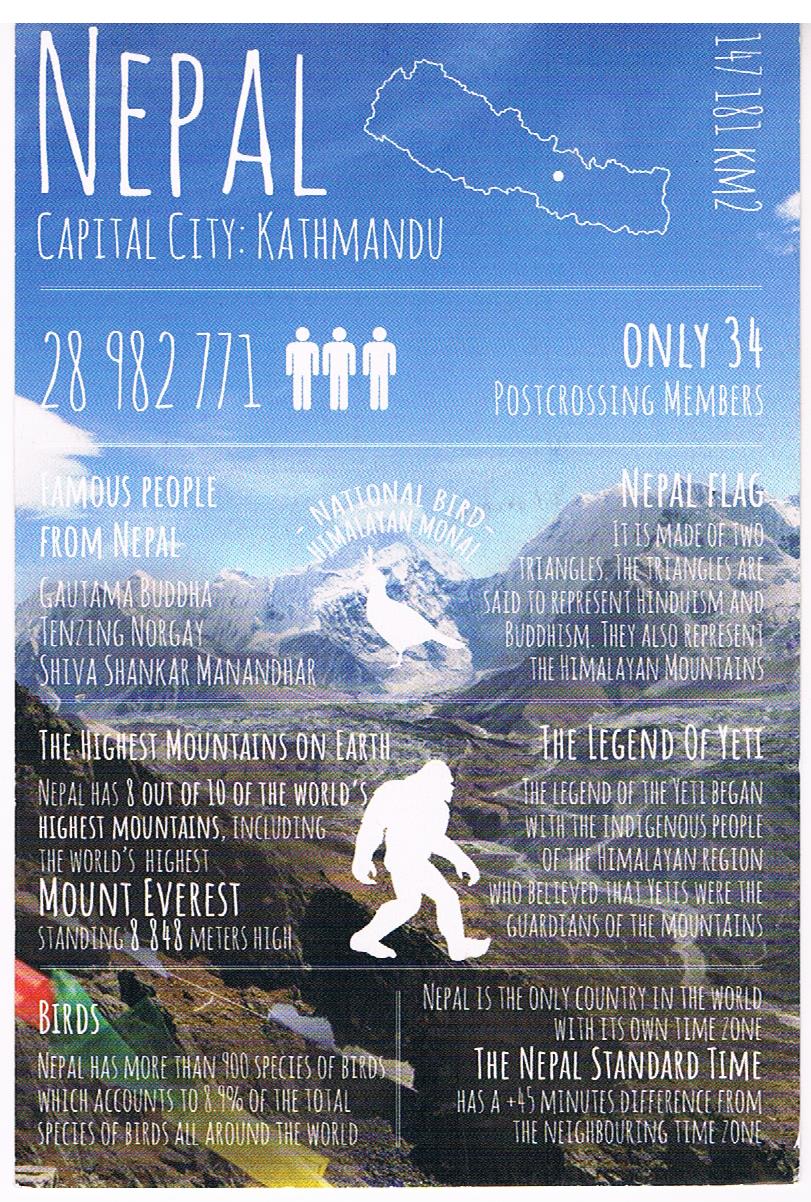This vertically aligned rectangular image appears to be an informative poster or flyer, likely aimed at promoting a trip to Nepal. The background features a stunning landscape with a clear blue sky, accented by a few white clouds, and a range of majestic, snow-capped mountains with a rocky foreground. 

In the upper left corner, in prominent white text, it says "NEPAL," next to an outlined map of the country. Beneath this, in smaller white text, it provides essential details: "Capital City: Kathmandu." Further down, it mentions the population of Nepal, marked as "28,982,771," accompanied by three iconographic human figures. To the right, it notes, "Only 34 post-crossing members."

A horizontal line divides sections of content. The next segment lists "Famous People from Nepal," including Gautama Buddha, Tenzing Norgay, and Shiva Shankar Manadhar. Adjacent to this is a mention of the Nepalese flag, followed by some right-aligned explanatory text.

Another line separates this from information about the "Highest Mountains on Earth," likely featuring details about the renowned peaks within the Nepalese Himalayas. On the right, it introduces "The Legend of Yeti," complete with an iconic image of a white-furred Yeti.

The bottom portion of the poster is divided into two sections: the left side elaborates on the diverse "Birds" found in Nepal, while the right side informs readers that "Nepal is the only country in the world with its own time zone," specifying that Nepal Standard Time is unique with a 15-minute plus 45-minute difference from neighboring time zones.